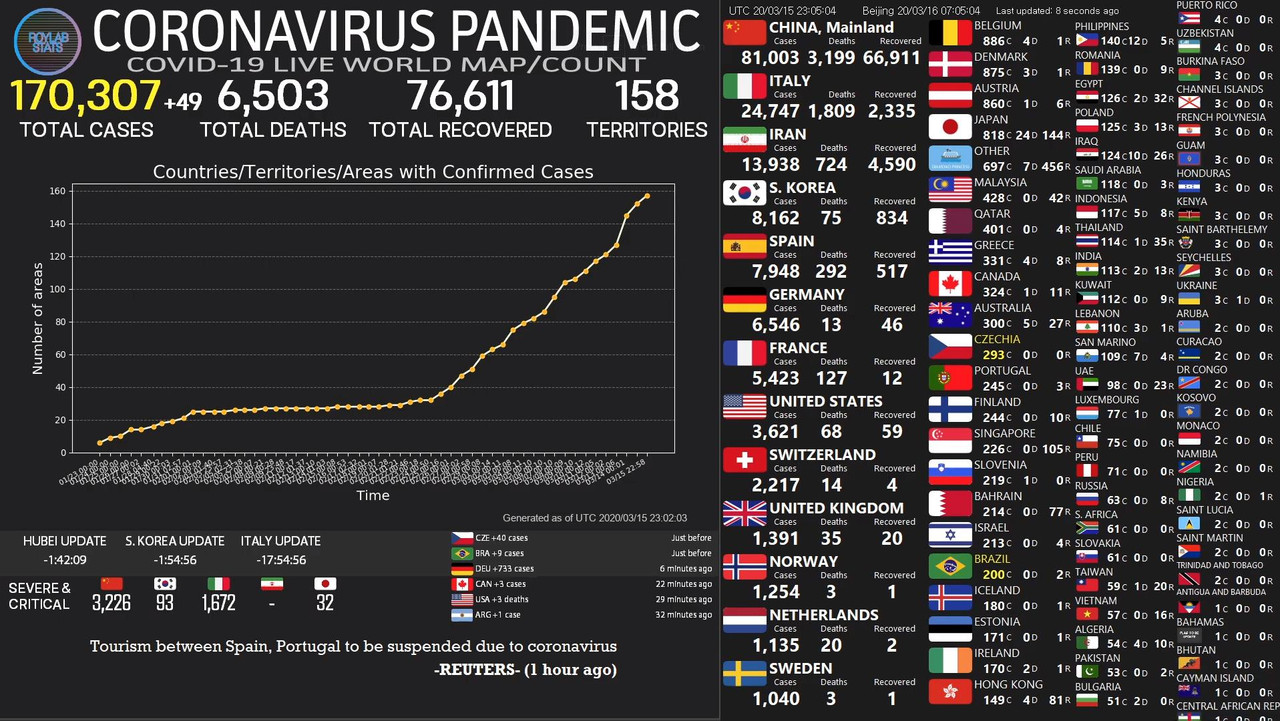This screenshot captures an early phase of the Coronavirus pandemic, displaying a live world map count labeled "COVID-19." At this point, there were 170,307 confirmed cases globally, with 6,503 total deaths and 76,611 recoveries across 158 territories. The image features a chart illustrating a rising death rate and notes that 3,226 cases were classified as severe and critical. It details the suspension of tourism between Spain and Portugal. 

A country-specific breakdown includes:
- China: 81,000 cases, 3,000 deaths
- Italy: 24,000 cases, 1,800 deaths
- Iran: 13,000 cases, 724 deaths
- South Korea: 8,000 cases, 75 deaths
- United States: 3,600 cases, 68 deaths

The detailed data underscores the rapid spread and escalating severity of the pandemic during its early stages.